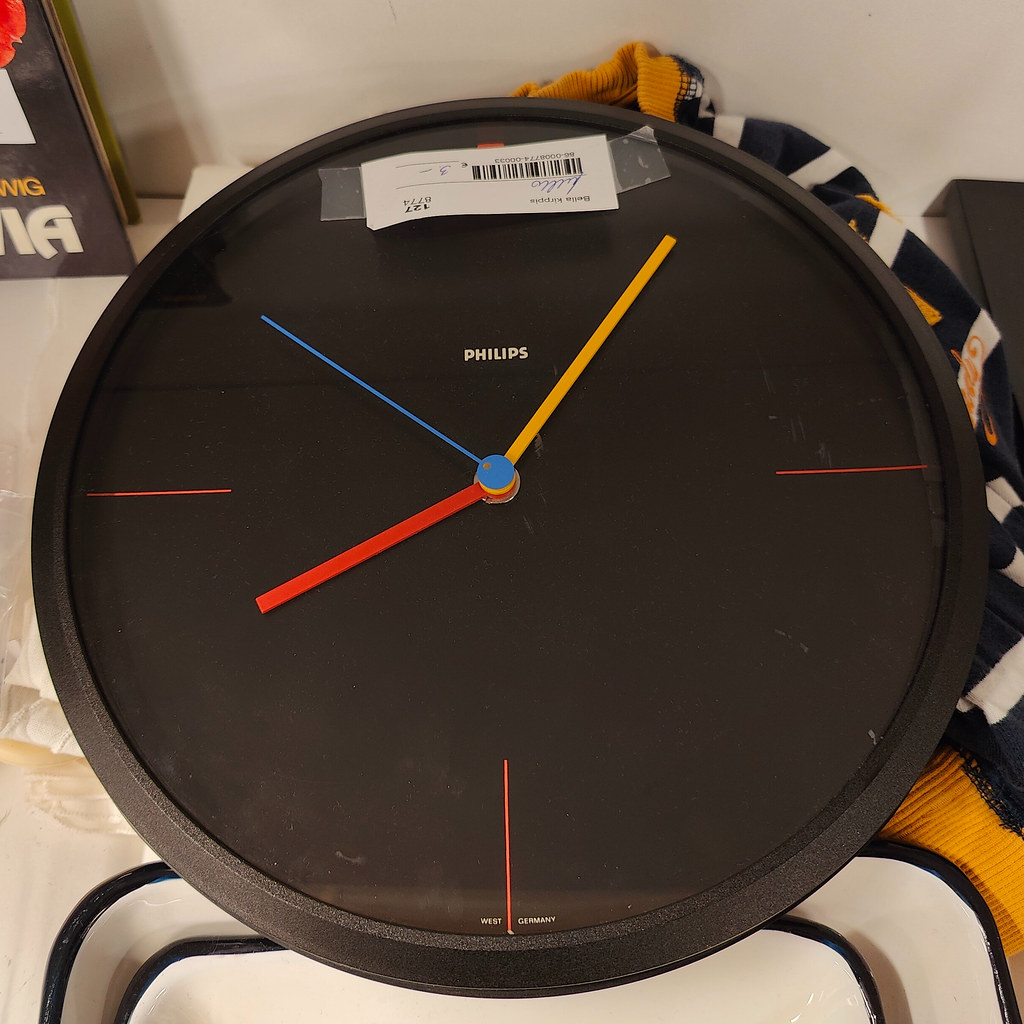This photograph features a large round black Philips wall clock resting horizontally on a beige surface. The clock's design includes a minimalist face with only four colored lines marking the 12 o’clock, 3 o’clock, 6 o’clock, and 9 o’clock positions. The 12 o'clock line is a thick red stroke, and the lines at 3, 6, and 9 o'clock are thinner red lines. The clock’s hands are vividly colored: the hour hand is bright orange, the minute hand is lemon yellow, and the second hand is a powder blue. The small white brand name "Philips" is positioned just below the 12 o'clock line. A white tag, secured with transparent tape and bearing a barcode and an upside-down signature, is affixed to the top of the clock face, indicating it might be sold or has been recently purchased. Surrounding the clock, there is a hardcover book situated in the upper left corner and what appears to be a striped garment underneath – possibly a blue and white sweater with an orange collar and trim. Additional items, possibly trays, are visible below the clock. The photo's background includes sections of both beige and white surfaces.